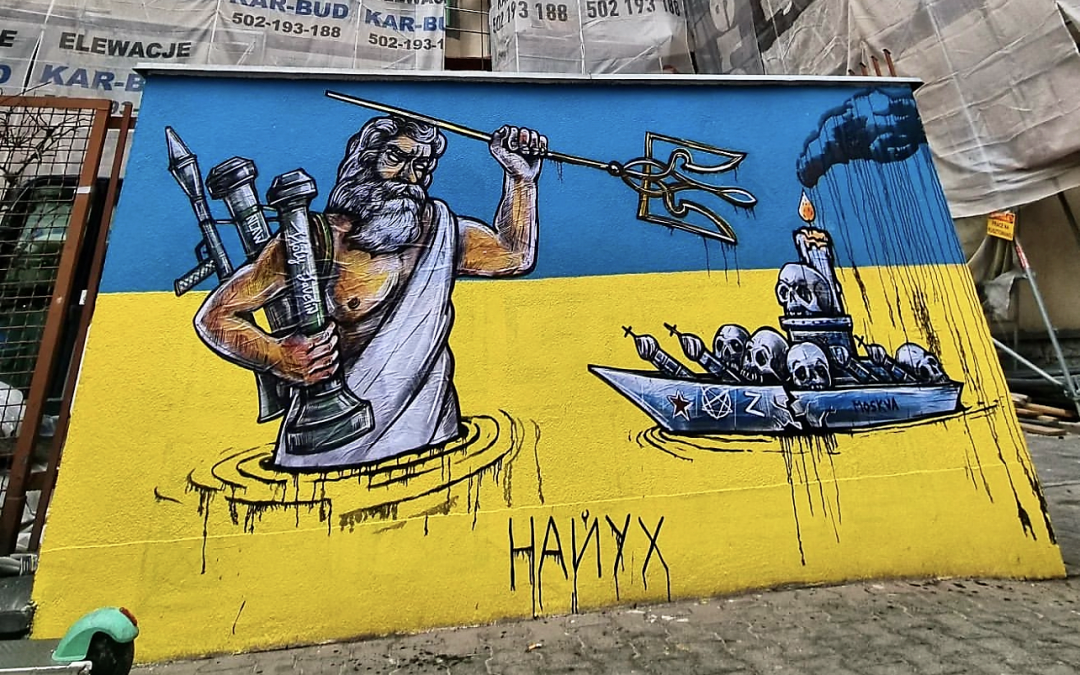A photograph captures a striking street scene where a large, detailed artwork leans against a gray cobblestone surface. Central to the image is a vivid painting set against a backdrop of blue and yellow, reminiscent of the Ukrainian flag—blue at the top and yellow at the bottom. The painting depicts a powerful sea god, possibly Poseidon, with white hair, beard, and a flowing Roman-style robe. Emerging from a yellow sea, he brandishes a trident towards a small, ominous boat filled with skulls and topped with a candle. Dark blue clouds above the boat appear to release black rain. Surrounding the scene are white signs and sheets of paper, one reading "Elevatia" and another with the repeated word "K-A-R-B-U-D" in blue font. At the bottom of the painting, the letters "H-A-N-Y-X" are scrawled in black, drippy spray paint, adding a dramatic finishing touch.